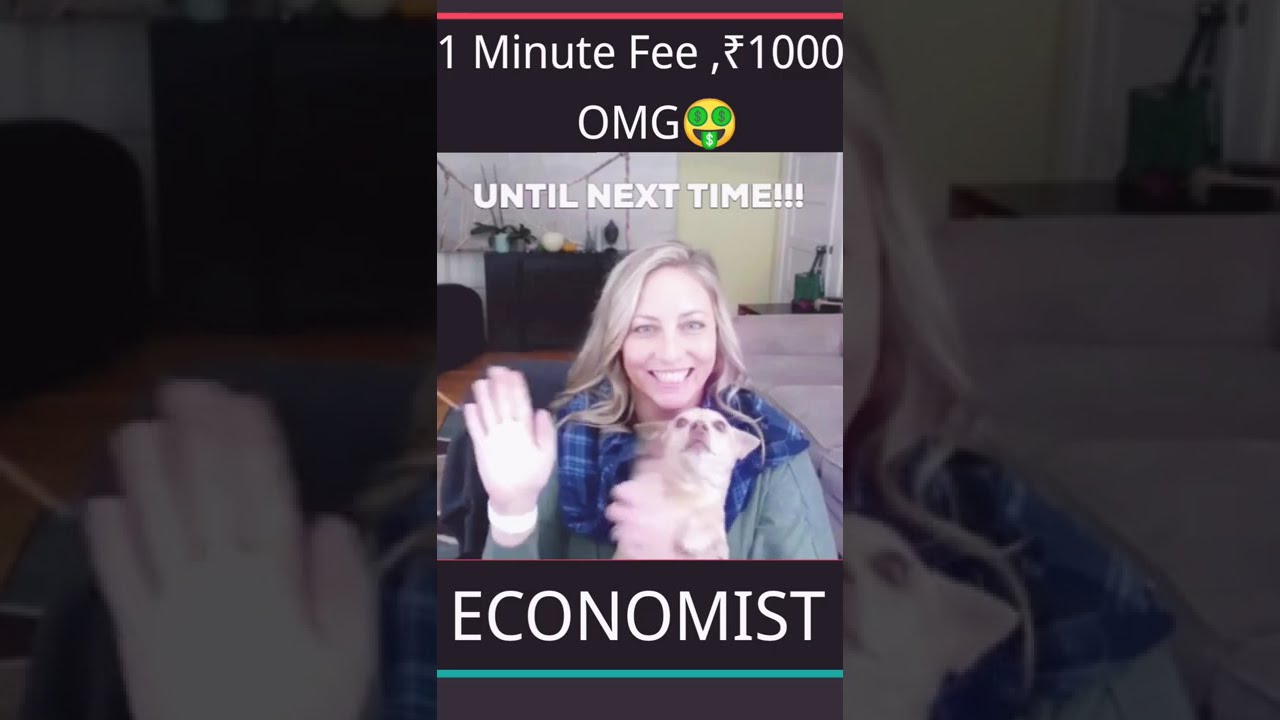The image appears to be a TikTok ad or a social media screenshot, designed in a smartphone aspect ratio. It depicts a white woman with long blonde hair, waving with her right hand, while holding a small chihuahua-sized dog in her lap. The woman's right wrist features a bracelet or wristband. She is dressed in a dark gray shirt complemented by a blue checkered scarf. The scene is set against a colorful backdrop, with darker borders framing the main content.

At the top of the image, the text reads: "One minute fee, 1,000," followed by "OMG" and the emoji with dollar signs for eyes and a tongue sticking out, also adorned with a dollar sign. Beneath this, the phrase "Until next time!!!" is displayed. At the very bottom, the word "Economist" is prominently featured in bold white capital letters, underlined with a blue-green line. Flanking the central image on the left and right are zoomed-in versions of the same picture, giving a sense of a portrait already captured on a cell phone, all within a landscape orientation.